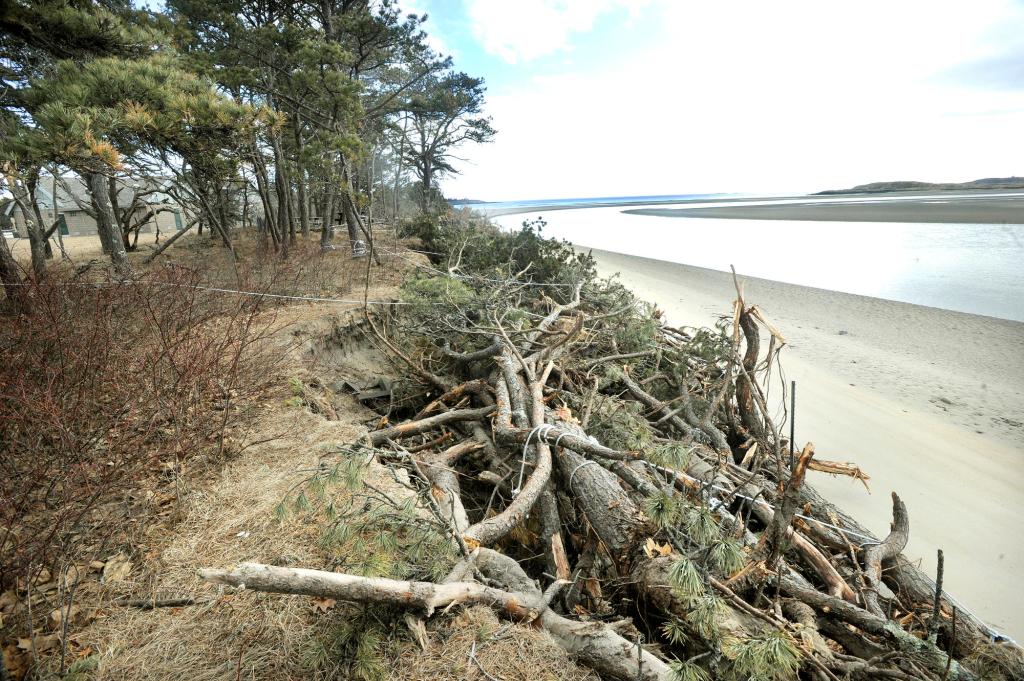The image portrays a picturesque coastal beach where a river meets the ocean. On the left side, a patch of trees, along with dried foliage and grass, gently frames the scene. To the right, a stream carves its path toward the distant ocean. Dominating the center of the image is a substantial pile of sticks and branches, meticulously strapped together and anchored by ropes tied to trees atop the beach bank. This arrangement appears to be an attempt to prevent beach erosion, with the lumber forming a barrier between the sandy shore and the area with trees and plants above. The beach's sand transitions from grey to a beige, softer texture, leading up to the extensive pile of branches. Peeking through the backdrop of tall trees standing atop the bluff, one can discern a building with a distinctive grey base, a green door, and a grey roof. Its architecture features a half-circle front and a pitched roof. The sky above is bright and heavily clouded, casting a reflective light on the water, adding to the serene atmosphere of this secluded coastal scene.